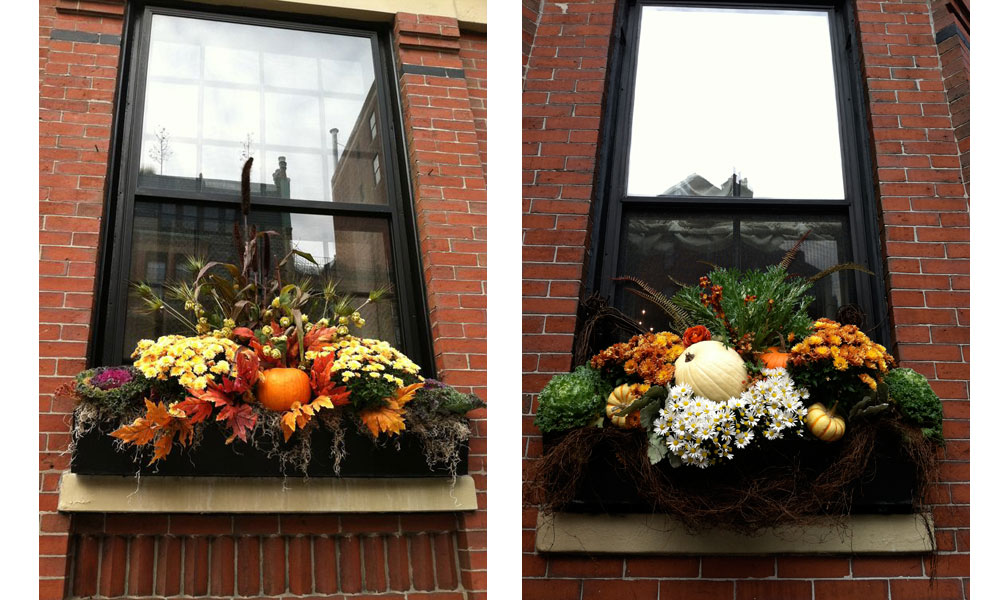In these two separate images, each depicts a square window on a red-bricked building with white-gray mortar. Both windows feature black frames and are adorned with flower planters hanging on the outside. The planters, which are black boxes, contain an array of artificial decorations including flowers, leaves, and vegetables, suggesting a seasonal or thematic decoration.

The left image showcases a fall or Halloween-themed arrangement, with vibrant colors including oranges, reds, greens, purples, and yellows. At the center, there is an orange vegetable, possibly a pumpkin, surrounded by yellow flowers, green leaves, and additional orange foliage, evoking a festive fall atmosphere.

The right image, while maintaining a similar aesthetic, shifts towards a Thanksgiving theme. It features a white circular fruit resembling a pumpkin at the center. This is accompanied by white and yellow flowers, a prominent red rose, and orange flowers complemented by green elements around the edges and top. A reflection of the city is faintly visible in the clean, darker windowpane, further enhancing the scene's ambiance.